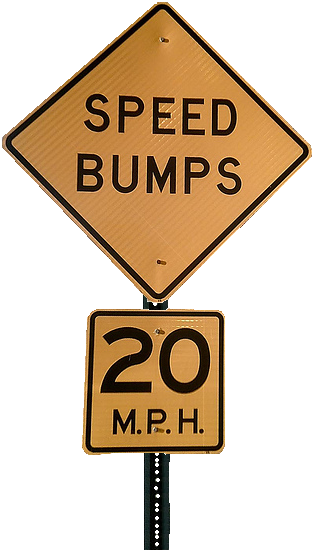The image depicts a close-up view of a traffic sign against a solid white background. The signpost is green metal, holding two clean, graffiti-free road signs. The top sign is a yellow diamond-shaped sign with a black border and bold black letters that read "SPEED BUMPS." Directly beneath it, there is a smaller square sign, also yellow with a black border, indicating "20 MPH." The white background is unbroken and featureless, emphasizing the traffic signs and their clear warnings of speed bumps and a speed limit of 20 miles per hour.